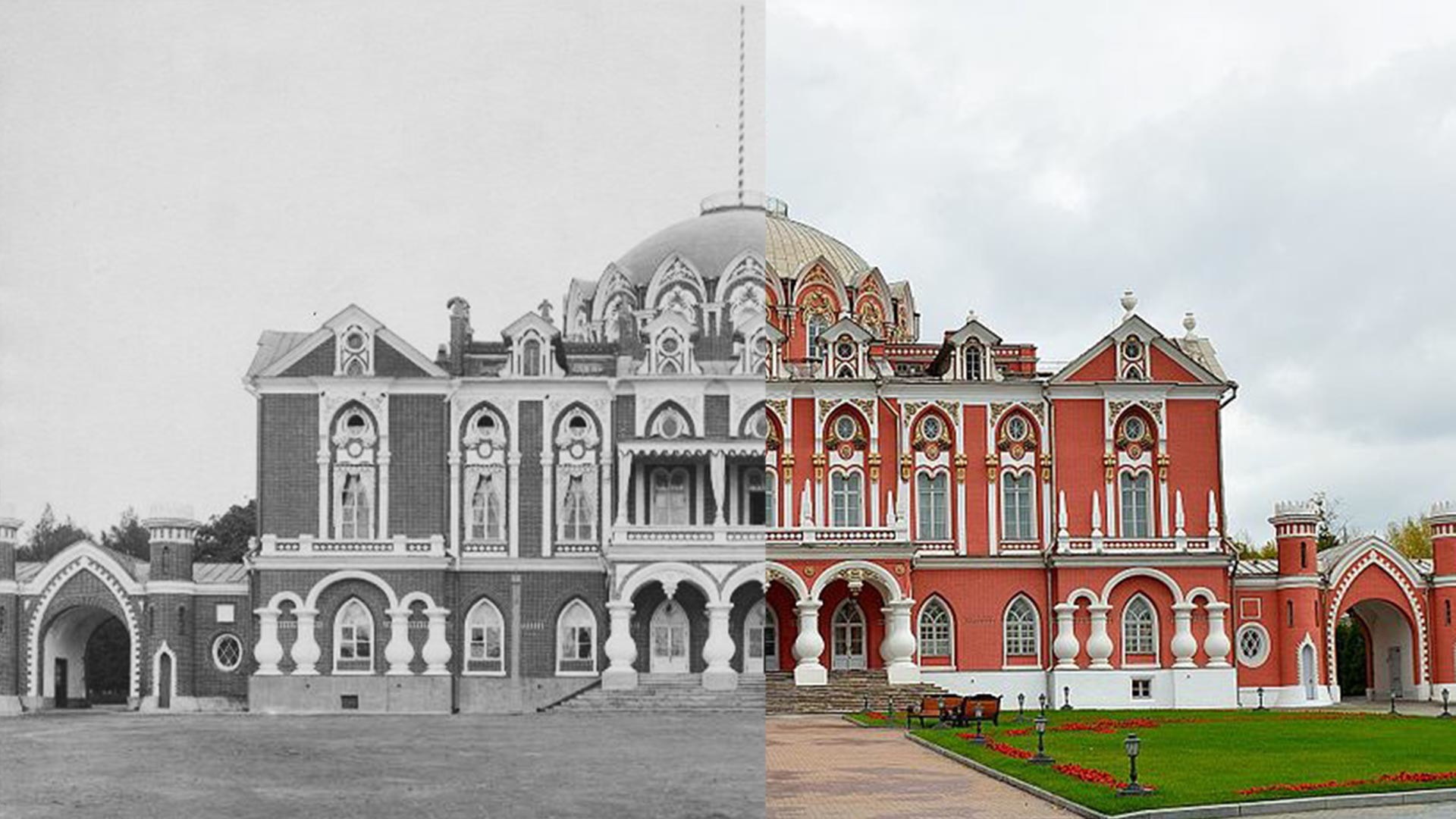The image depicts a grand, historic building, divided perfectly down the middle into two contrasting halves. The left-hand side of the image is an old, black-and-white photograph, offering a glimpse into the past. This side reveals a large, ornate structure with cathedral-style windows, intricate white arches, and a prominent dome atop the edifice. It's evident that this is either a palace or a university building from another era. The right-hand side of the image presents the same building in vibrant color, showcasing its current, restored state. The building itself is a rich blend of salmon, reddish-brown, and orange hues, with pristine white trim. The modern half also features a green lawn adorned with red flowers, set against a backdrop of a gray sky. Notably, there are multiple arches within the structure, including two large arches at each end, serving as entryways to a courtyard with smaller turrets, and three central arches that likely function as doorways. This juxtaposition of the black-and-white past and the colorful present highlights the building’s majestic architecture and its preservation through time.